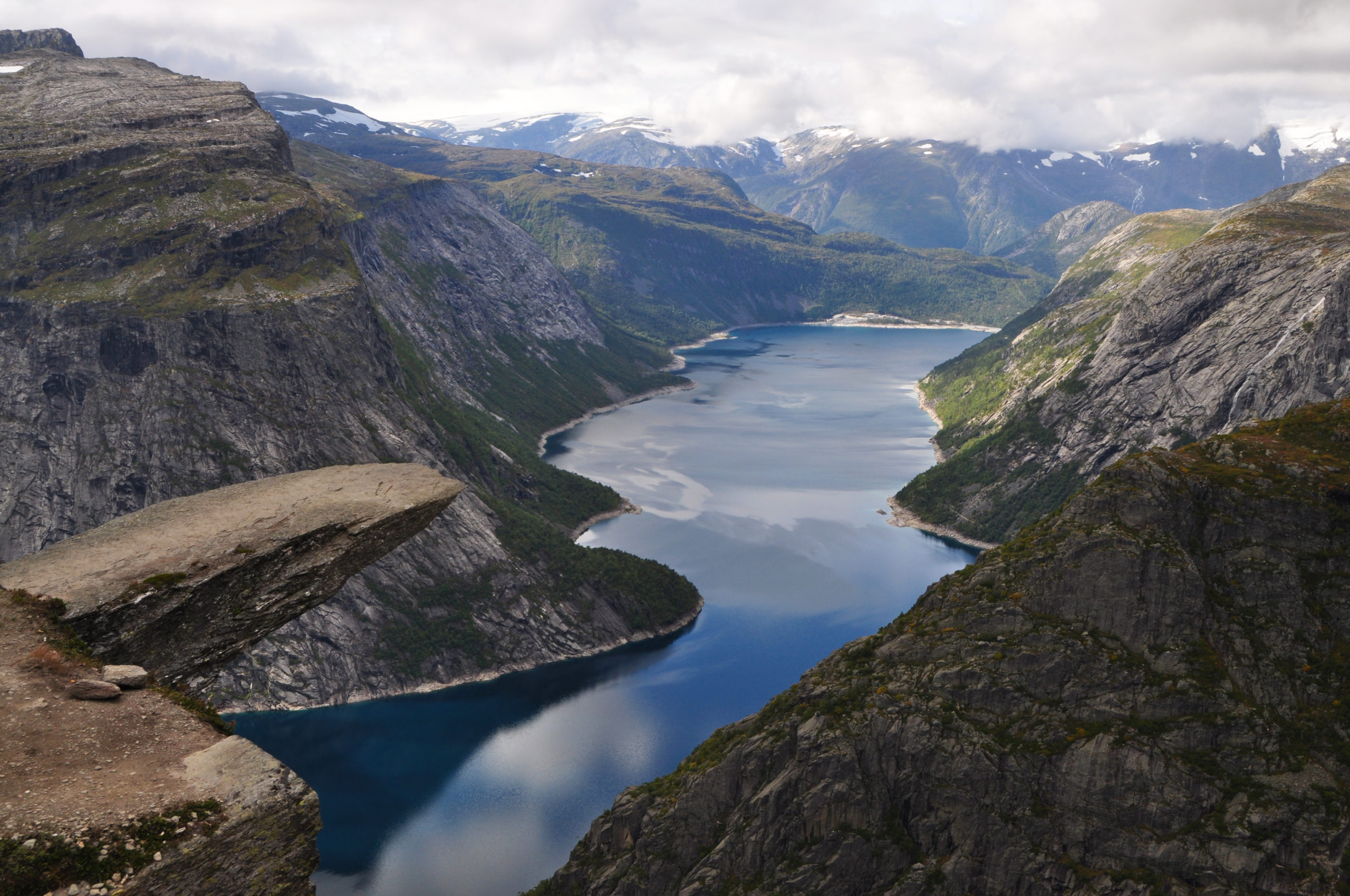This image displays a breathtaking canyon landscape that seems to be taken from an aerial perspective, possibly from an airplane. The expansive crevice houses a strikingly blue river or creek that winds through the scene. Surrounded by steep, brownish rocks adorned with patches of green from either algae or small trees, the rugged terrain appears perilous yet splendidly captivating. The background is graced by towering, snow-capped mountains, beneath a sky scattered with clouds. The clouds cast reflections on the river’s surface, adding a surreal touch to the composition. Though the photo is very zoomed out, it offers a comprehensive view of the picturesque setting, accentuating the contrast between the verdant greens, earthy browns, and the deep, tranquil blue of the water. The entire scene is bathed in natural beauty, showcasing an awe-inspiring place for sightseeing, reminiscent of landscapes found in states like Utah.